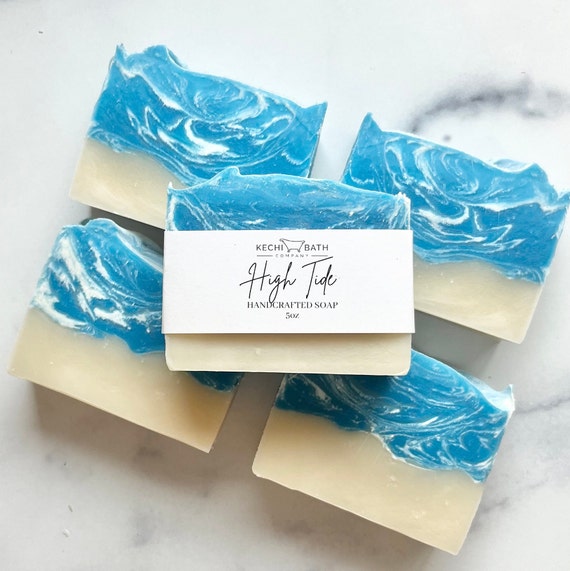This is an extreme close-up overhead photograph of five handcrafted bars of soap, perfect for showcasing on Etsy, Instagram, or a product website. Four of the bars are arranged in a square pattern on a white marble table with subtle black streaks. Each soap bar features a creamy ivory white base with the top half displaying an aqua blue hue interlaced with intricate white swirls, resembling a white and blue swirl fudge. The fifth bar sits on top of the others, prominently displaying a label that reads "Keech Eye Bath Company." The label includes an illustration of a bathtub and notes that the soap is "High Tide Handcrafted Soap," weighing five ounces. The soap's rectangular shape with jagged edges and unique color pattern gives it an upscale, artisanal appearance, making it a striking and elegant product.